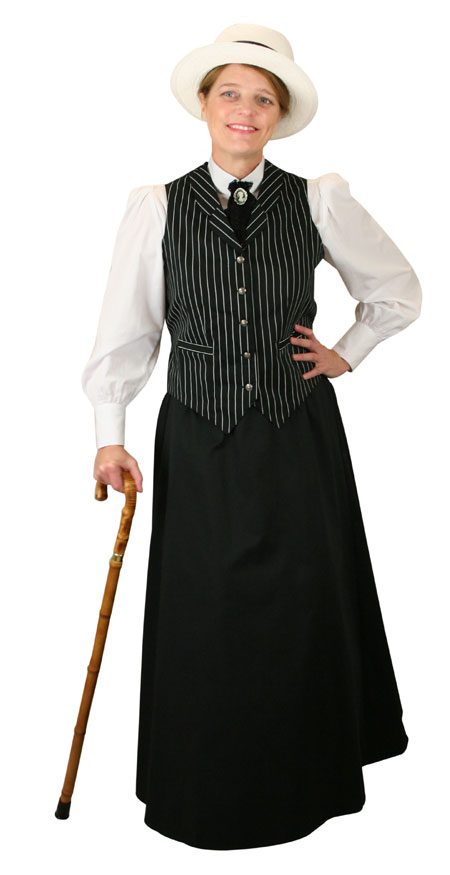The image features a woman dressed in a vintage-inspired Mary Poppins-like outfit, standing against a stark white background. She is facing the camera with a slight smile, revealing a hint of her teeth and her red lips. Her attire includes a long black skirt reaching down to the floor and a black and white pinstripe vest fastened by five silver buttons. Beneath the vest, she wears a white, poofy-sleeved blouse with a high collar, adorned with a black tie secured by a cameo pendant. On her head rests a slightly tilted white straw hat with a visible black hat band, offering a glimpse of her short, reddish-brown hair. In her right hand, she holds a bamboo cane with a brass ring near its black tip, while her left hand is placed on her hip, her fingers visibly relaxed. The woman evokes a sense of timeless charm, striking a poised and confident stance as she looks slightly off into the distance.